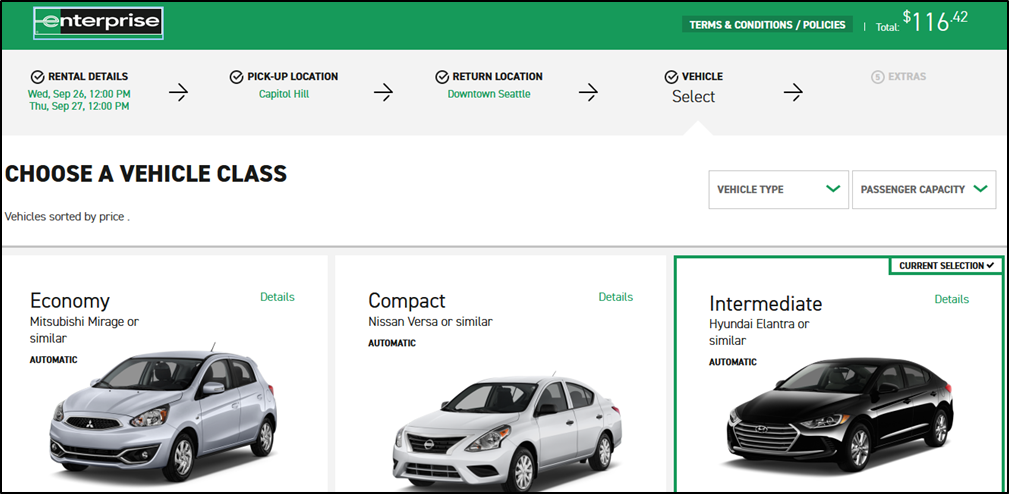This image is a screenshot from the Enterprise car rental website. In the top left corner, the Enterprise logo is prominently displayed. At the top of the screen, a thin green navigation bar contains links, with "Terms and Conditions/Policies" visible on the right. To the far right of this bar, the total rental cost is listed as $116.42.

Below the navigation bar, there is a large box with a grey background that contains detailed rental information. On the left side of this box, the rental details are outlined, which include the rental period: from 12 PM on Wednesday, September 26th to 12 PM on Thursday, September 27th. The pickup location is specified as Capitol Hill, and the return location is Downtown Seattle. Additionally, there is a section labeled "Vehicle Select" with an arrow next to it, and a note in light grey below it.

In the next section of the screenshot, the title "Choose a Vehicle Class" is presented. Adjacent to this title are two dropdown boxes labeled "Vehicle Type" and "Passenger Capacity."

Below this section, three car options are displayed. On the left is the Economy option, represented by a Mitsubishi Mirage or a similar automatic vehicle. In the center is the Compact option, showing a Nissan Versa or a similar automatic vehicle. On the right, the Intermediate option is highlighted, featuring a Hyundai Elantra or a similar automatic vehicle. The Intermediate option is marked with a "Current Selection" tag in the upper right-hand corner.

The image concludes with the phrase "Thanks for watching!"